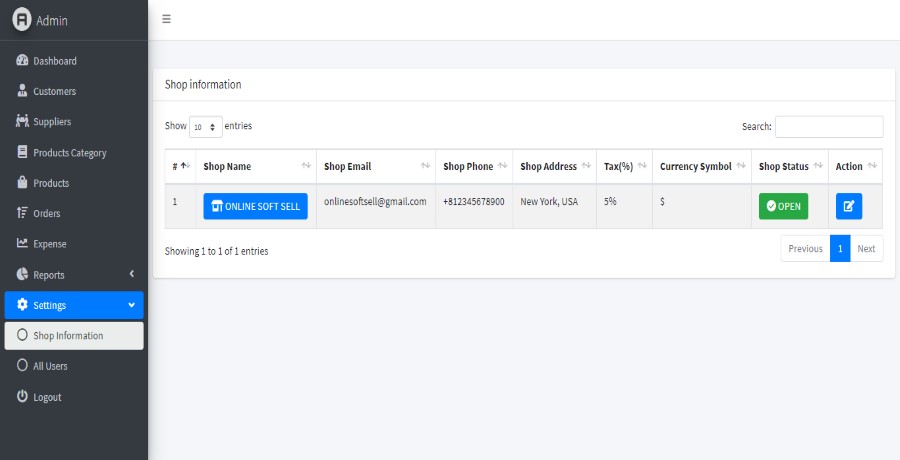**Admin Control Panel Overview**

On the left side of the webpage, a tall, rectangular admin control panel spans from top to bottom. At the top, the word "Admin" is displayed prominently next to a white circle containing the letter "A." Below, several navigational options are listed vertically: Dashboard, Customers, Suppliers, Product Categories, Products, Orders, Expense, and Reports. A blue rectangular box labeled "Settings," accompanied by a gear icon, follows Reports. Beneath this, a white box displays "Shop Information." Further down, on a dark blue or dark gray background, options for "All Users" and "Logout" are visible.

To the right of the control panel lies the main webpage content. At the top, the heading "Shop Information" precedes a detailed graphical chart with several categorized sections: Shop Name, Shop Email, Shop Phone, Shop Address, Tax Percent, Currency Symbol, Shop Status, and Action. Each section is filled in with various corresponding details, comprising numbers and text that provide specific information about the shop.